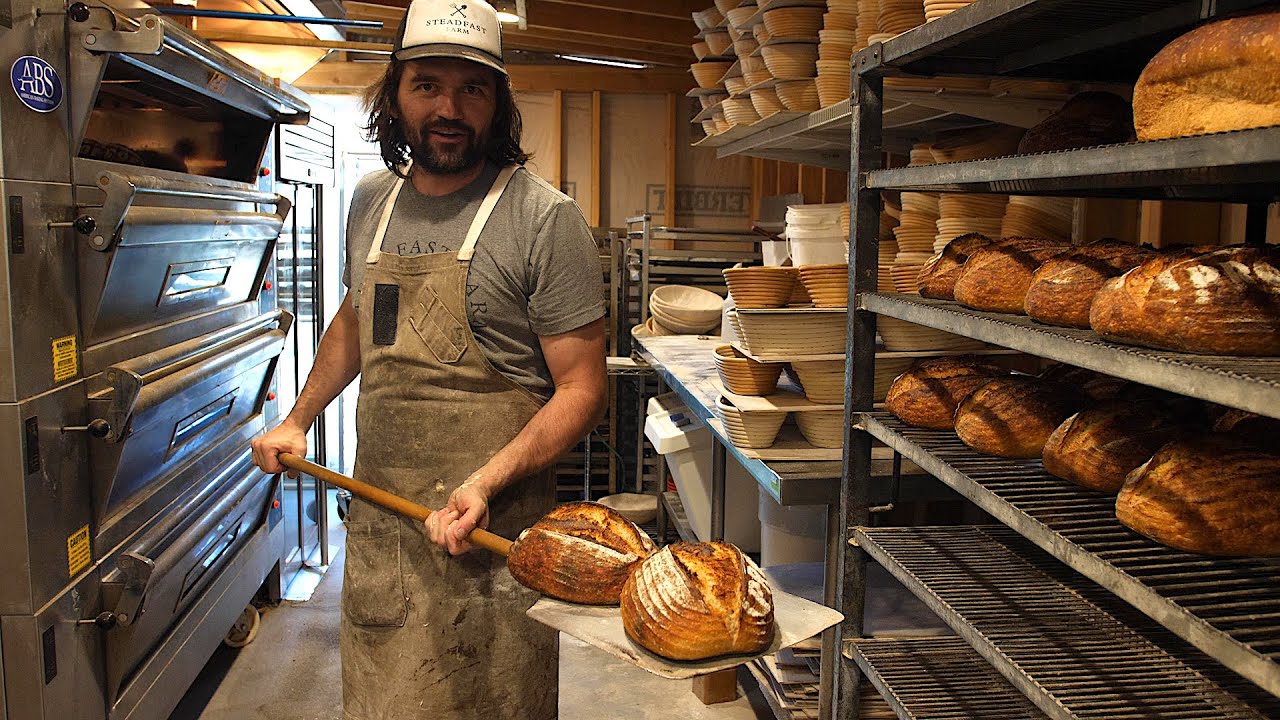In the bustling back room of a bakery, a bearded man with long brown hair stands in the center, encapsulating the spirit of artisanal bread-making. Clad in a weathered leather or waxed canvas apron over a gray t-shirt, and wearing a baseball cap emblazoned with the word "Steadfast," he grips a long, wooden bread slide. This paddle-like tool, designed for maneuvering bread in and out of ovens, holds two freshly baked, golden-brown loaves, likely sourdough, still steaming from the heat.

The left side of the frame is dominated by large pizza ovens with doors that swing open downward, ready to bake another batch. On the right, several metal shelves are visible, stacked with a mix of round loaves, some racks full while others are waiting to be utilized. Between the man and the cooling racks, there's a cluttered preparation area featuring various kitchen bowls of different sizes, a marble counter, and even a washer tucked underneath. Above, additional shelves are filled with colorful pots, adding a splash of vibrancy to the busy, utilitarian space. This vivid kitchen scene captures a moment in the life of a dedicated baker, diligently moving loaves from the oven to the cooling rack, surrounded by the essential tools and ingredients of his trade.